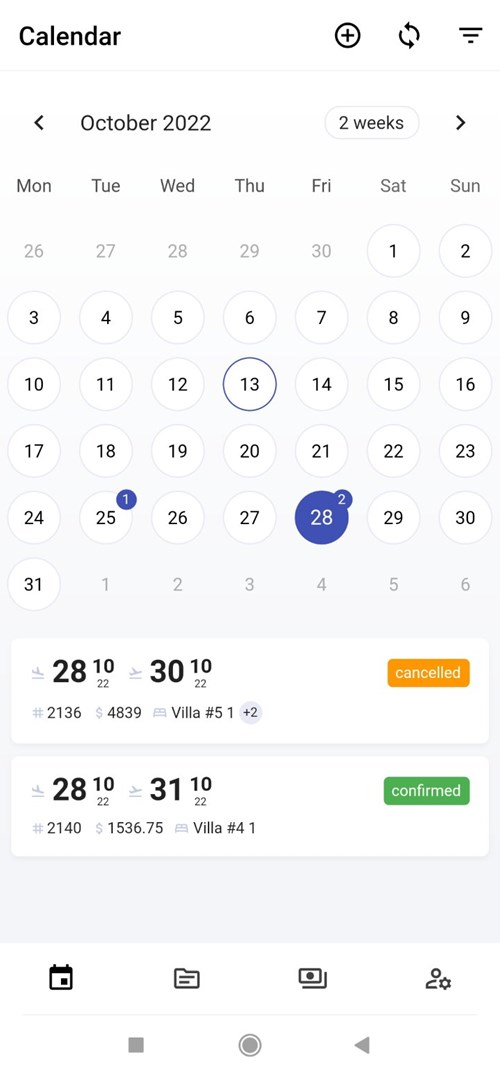The image appears to be a screenshot from a mobile device, likely a cell phone or tablet, given the aspect ratio and the presence of familiar icons. In the upper corner of the screenshot, there is what appears to be a Wi-Fi signal icon. At the bottom, the screen displays the typical navigation icons seen on Android devices: the back button, home button, and the recent apps button.

The interface shown in the screenshot belongs to a Calendar application. The top section of the app features the word "Calendar" in black text, set against a primarily white background. Adjacent to this title are three icons: a plus sign for adding new events, a refresh icon, and another icon that appears to represent signal strength.

Directly below this header are the words "October 2022" followed by a bubble stating "2 Weeks". The calendar view below lists the dates, with October 28th highlighted in blue and marked with a number "2" bubble above it. Similarly, October 25th has a number "1" bubble. Additionally, the 13th is outlined with a blue line.

At the bottom of the screen, there are event details for October 28th. One entry lists "28 10:30 to 10:30, villa number 5" and another entry for the same date and time lists "villa number 4". The first entry has an orange "Canceled" button, indicating it was canceled, while the second entry has a green "Confirmed" button, indicating it was confirmed.